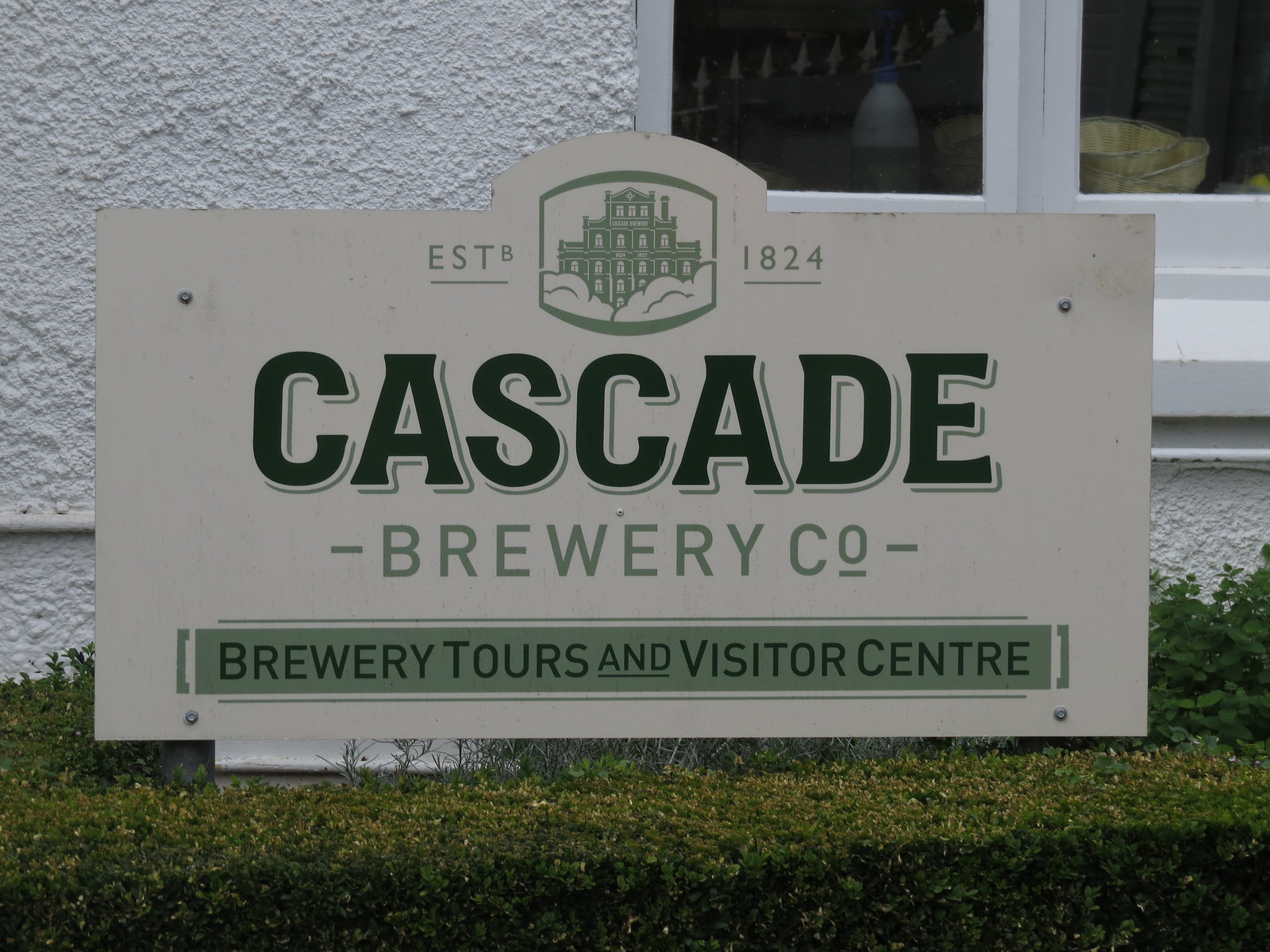This photograph captures a professional sign in front of a stuccoed building, featuring a detailed emblem of a historic-looking structure. The sign, predominantly white with various shades of green lettering, reads "ESTB 1824" at the top, flanked by the green emblem. Below, in bold darker green, it says "Cascade," followed by "Brewery Company" in a lighter green font. At the bottom, on a green strip with dark green letters, the sign promotes "Brewery Tours and Visitor Center." The sign is mounted on a support structure emerging from dense green shrubbery. The background building has a white stucco finish with visible windows that provide a glimpse of bottles, wicker baskets, and light fixtures inside. A hint of blue can also be seen in the picture, adding a subtle contrast to the dominant grey, white, and green tones.